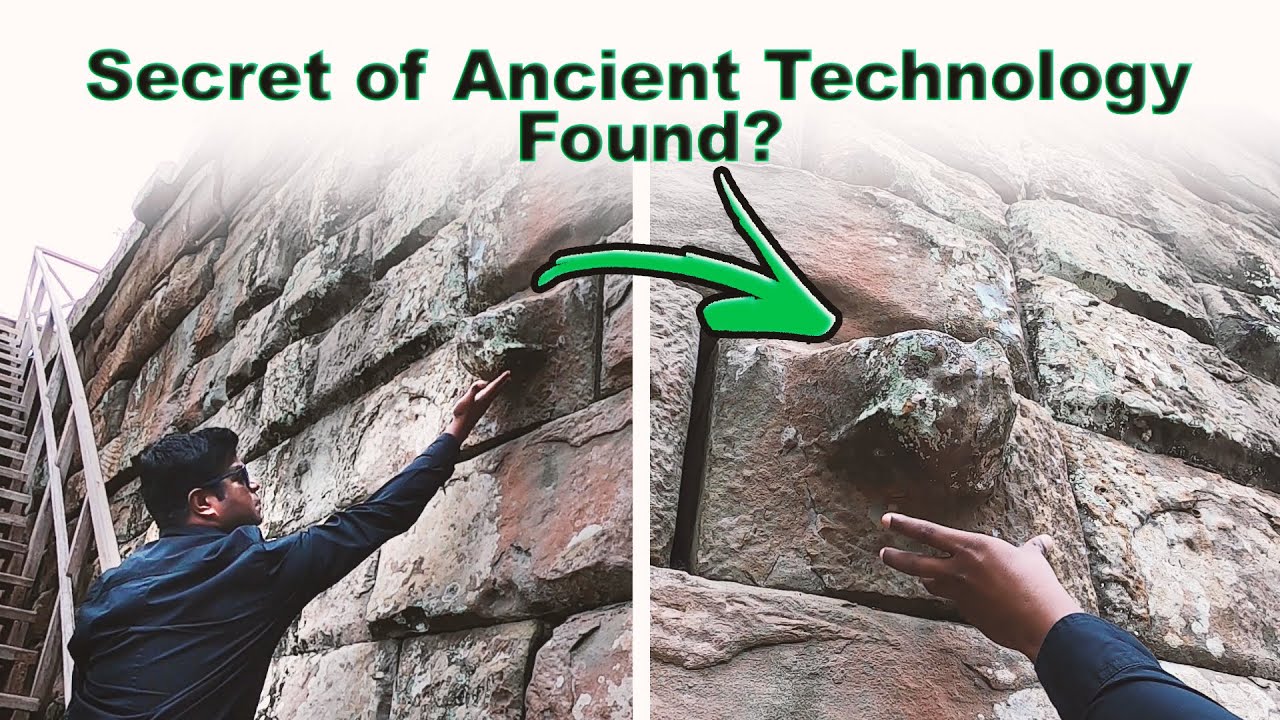The image consists of two photos placed side-by-side, both featuring a man interacting with an ancient stone wall. The text above the images reads "secret of ancient technology found?" in green text, with each word capitalized except "found."

In the left photo, the man, who appears to be of Asian descent, with dark black hair and black sunglasses, is reaching up toward a large, protruding stone on the wall. He is wearing a navy blue long-sleeve shirt. The stone wall is built from roughly rectangular, irregularly shaped rocks, arranged in about eight layers. There is a stairway with a white railing visible to the left of the man, leading from the base to the top of the wall.

The right photo provides a close-up view, focusing on the man's hand grasping the protruding stone, which is irregularly shaped and somewhat lumpy, possibly hinting at the "secret technology" referred to in the caption. The wall's texture and the stone's unique shape are clearly visible in this detailed shot.

The dual-image format highlights both the context of the man's interaction with the wall and a closer examination of the stone, adding depth to the mysterious claim suggested by the caption.